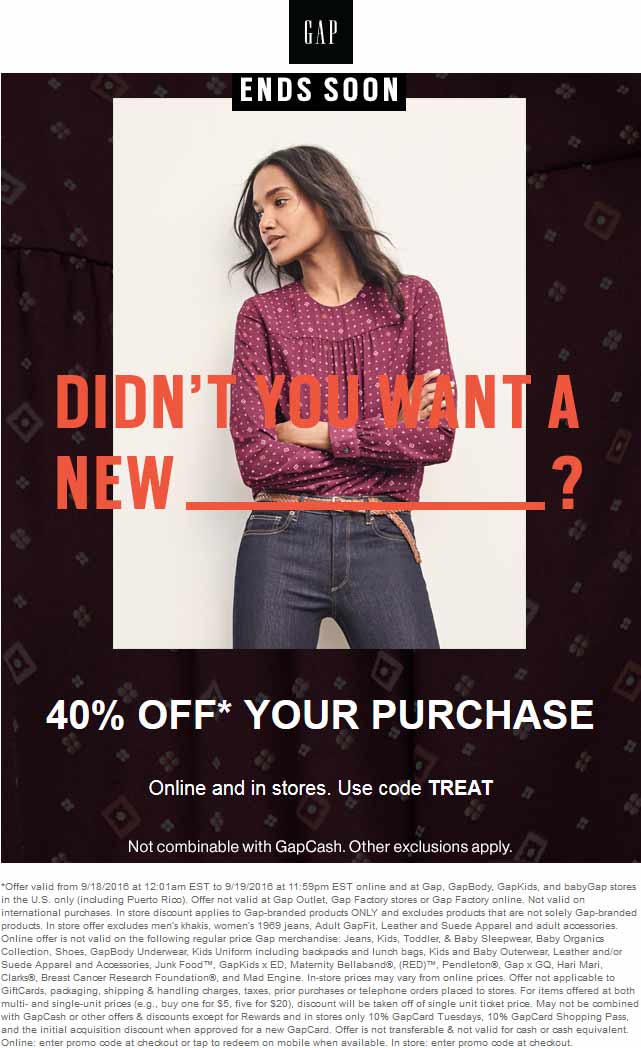In this image, there's an advertisement featuring a detailed design and promotional text. At the very top, a black square logo with the letters "GAPH" prominently displayed in white capital letters catches your eye. Underneath this logo, a large, tall, rectangular box dominates the composition.

The background of this box is a rich brown, adorned with a sophisticated pattern of gray and light brown floral and square paisley designs. These motifs add a touch of elegance and complexity to the backdrop.

Positioned slightly towards the top center of this background, there is an image of a woman. She is depicted with shoulder-length, wavy brown hair styled in a natural, casual manner. She's wearing a loose-fitting, long-sleeved shirt that is a blend of reddish and purplish hues. The shirt features the same square and flower paisley patterns in a subtler design, with buttoned wrist cuffs adding a refined detail. She pairs this top with tight blue jeans secured by a brown belt. The woman’s pose is relaxed, with her hands crossed at her lower waist, and her head is turned gently to the side, exuding a sense of ease and confidence.

This image of the woman is set against a light tan background, creating a clear contrast. Above her image, in a black rectangle with white font, the text reads "N soon." Overlaying her midsection, where her crossed hands are, orange text poses the question, "Didn't you want a new ____?" with a long underscore and a question mark, inviting viewers to fill in the blank.

Beneath her image, the brown background continues, providing a canvas for the promotional text. In bold white letters, it advertises "40% off*" and "your purchase." Below this, in smaller white text, it specifies, "online and in stores, use code TREAT," with "TREAT" boldly capitalized. Further fine print indicates that the offer is "not combinable with Gap Cash, other exclusions apply."

The very bottom of the advertisement features a large white box filled with a lengthy paragraph of small text detailing the terms and conditions of the promotion, ensuring all necessary legalities and restrictions are clearly communicated.